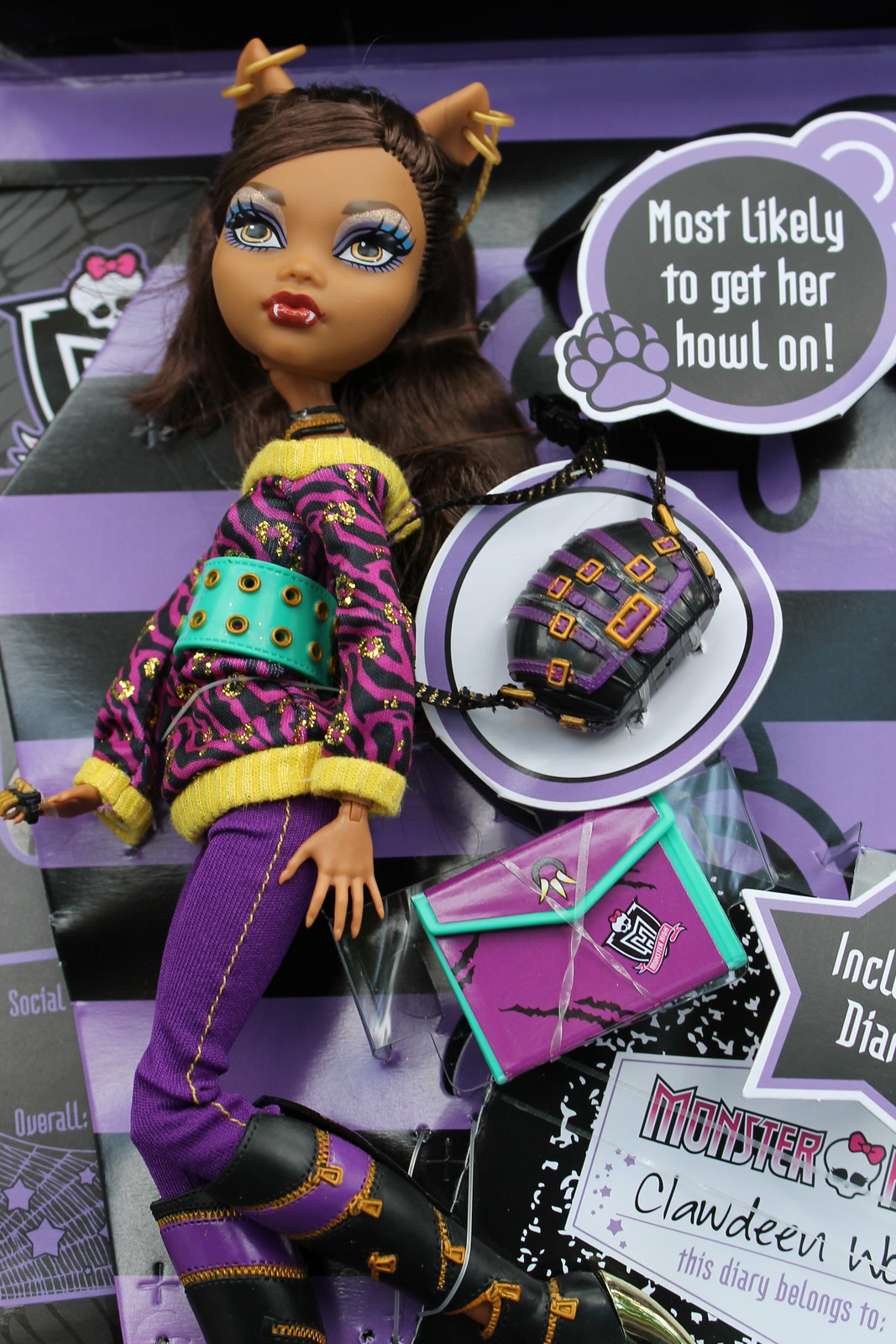The image showcases a detailed close-up of a Monster High doll named Claudine, specifically designed to resemble a werewolf character. Claudine has a dark complexion and is adorned with long, brown hair, sporting distinctive cat-like ears and fangs subtly protruding from her bottom lip. Her makeup is meticulously applied, accentuating her fierce look. She is dressed in a striking outfit consisting of a purple and black leopard print sweater with yellow cuffs, complemented by a turquoise belt with double divots. She wears purple jeans and a pair of elaborate boots that feature black, purple, and orange hues with gold designs. 

The doll is accessorized with a matching black and purple purse and possibly a helmet, adding to her ready-for-action appearance. Claudine's belongings are spread out against what seems to be a purple and black striped background, reminiscent of a tablecloth or gift wrap. To the right side of the image, there are bubbles with text, one of which reads, "Most likely to get her howl on" inside a paw print. Below it, there is another bubble containing her purse. The packaging prominently features the Monster High branding and a diary stating, "This diary belongs to Claudine." The scenario suggests that she is a popular toy intended for young children, standing out with her vivid colors and fierce aesthetic.